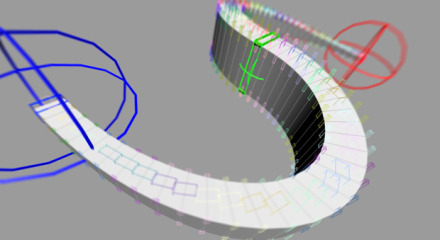The image depicts a 3D, S-shaped racetrack reminiscent of Rainbow Road from Mario Kart, but instead of being vibrantly colored, it is entirely white, giving it an unfinished appearance. This winding pathway, composed of rectangular sections that resemble piano keys, stretches out and scrolls downward in a serpentine form. The track is set against a black background and is flanked on each side by faintly colored lines representing the X and Y axes, commonly seen in 3D modeling software like Blender, in blue and red. Near the lower left end of the track, a large blue circle is visible, while the upper right end features a red circle. A small distinct green section and some gray areas are also present, adding subtle details to the scene.